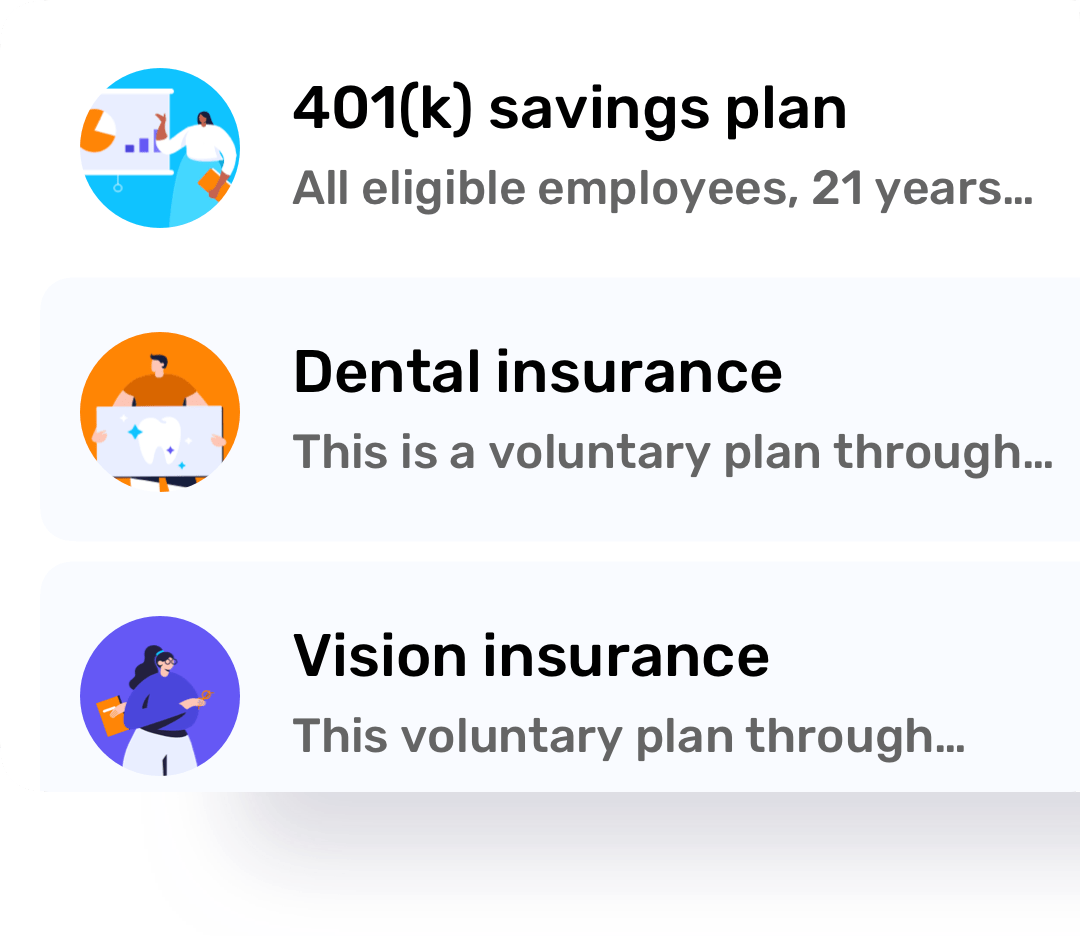This digital image is divided into three informative sections, each providing details about different employee benefits.

At the top, the first section features a white background within a rectangular shape. On the left side, there is a bright blue circle with a simple cartoon icon on it. The cartoon depicts a person with a very small head and brown skin, holding up an arm in front of a chart that includes an orange pie chart on the left and a purple bar chart on the right. To the right of this icon, in bold black text, it reads "401k Savings Plan." Beneath this, in dark grey text, it states, "All eligible employees 21 years..."

The second section below has a rectangle with a very light grey background and rounded corners. Similar to the first section, there is an icon on the left side, contained within an orange circle. The cartoon figure here is holding up a bluish piece of paper that features an illustration of a tooth, adorned with blue, white, and purple sparkle symbols. To the right of this icon, bold text reads "Dental Insurance." Underneath this, in dark grey text, it says, "This is a voluntary plan through..."

The final section has a very light blue background. The icon in this part includes a purple circle with a cartoon person standing on it, holding glasses in one hand and a book in the other. To the right of this icon, in bold text, it reads "Vision Insurance." Beneath this, in dark grey text, it mentions, "This voluntary plan through..."

This detailed description highlights the visual elements and the minimal text content of each section, proving a comprehensive overview of the information presented in the image.